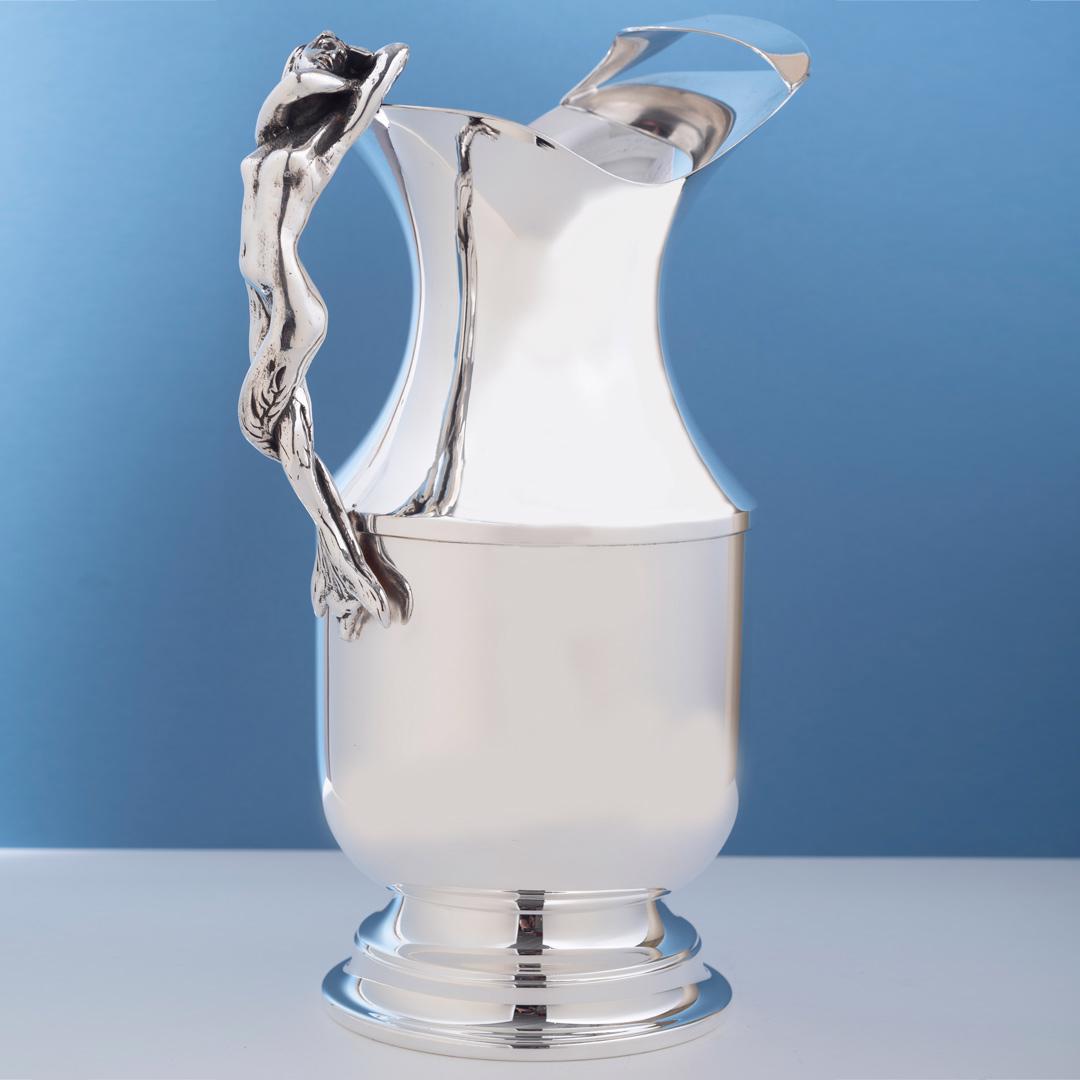The image features an elegantly designed metal pitcher or vase, crafted with high precision and potentially photographed or digitally created to mimic a photograph. The background is predominantly a calm, medium blue with the bottom eighth depicting a light gray surface reminiscent of a countertop. The pitcher, likely fashioned from highly polished chrome or reflective crystal, exudes a brilliant, almost glowing white sheen. Its intricately twisted, hand-forged-looking handle adds to the ornate appearance, with the reflective surface capturing its own handle’s image. The body of the pitcher is traditional in shape, with a multi-layered base in varying shades of silver, enhancing its sophisticated and timeless aesthetic. The spout is distinctive, designed uniquely to facilitate pouring. This beautifully elaborate container might be something cherished as a family heirloom or gifted on special occasions, symbolizing its grandeur and sentimental value.